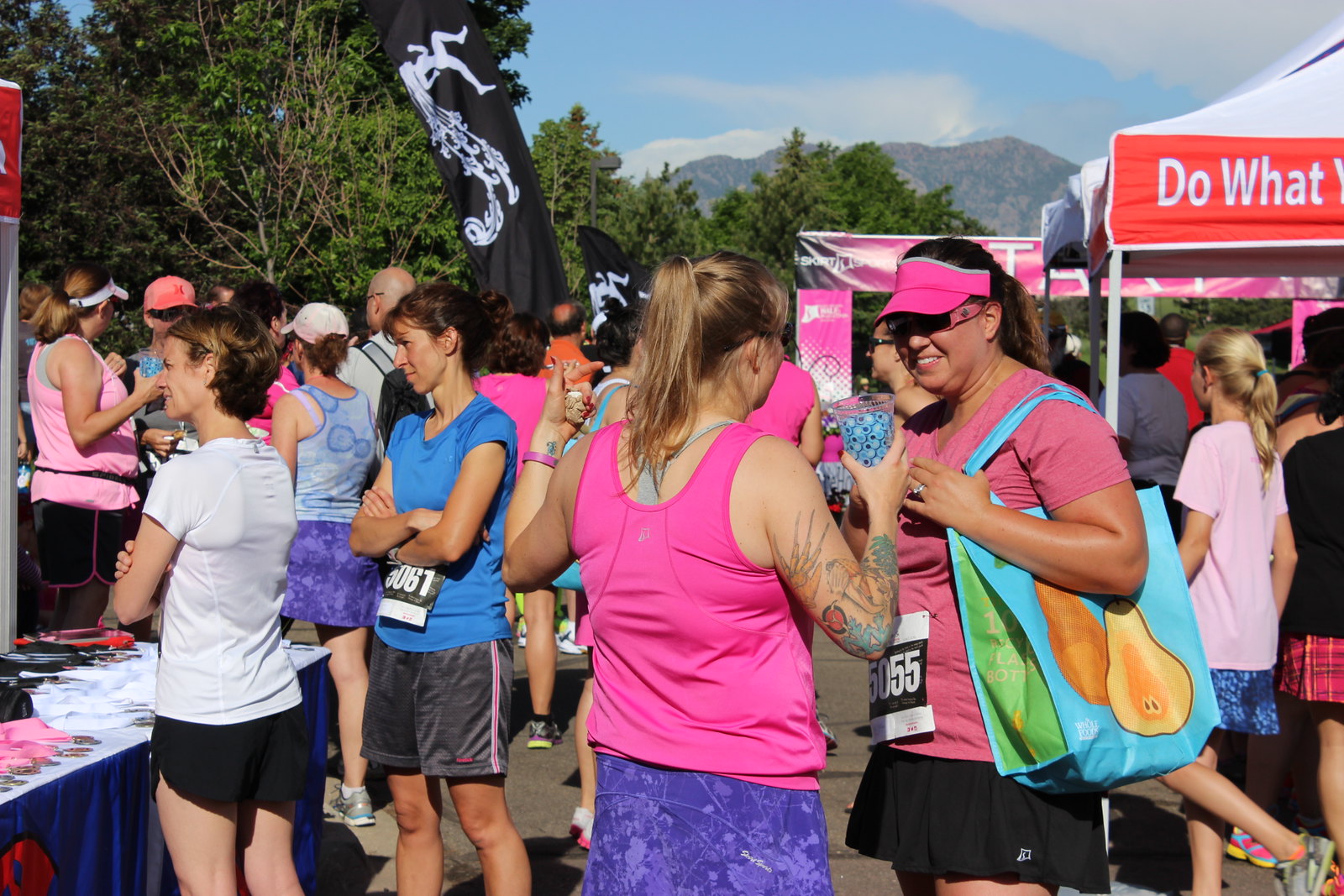This image captures a lively outdoor event, likely a breast cancer awareness marathon or race, characterized by a sea of participants dressed predominantly in pink. The foreground features two women: one with a pink tank top and purple shorts, identifiable by her blonde ponytail, fair skin, and extensive tattoos on her right arm and back. She is conversing with another woman in a pink t-shirt and visor, dark sunglasses, and a noticeable blue tote bag over her shoulder. Both women appear to be engaged in conversation, with the first woman holding up a glass or cup.

To the left, a pair of women stand near a registration or display table. One wears a white t-shirt and black shorts, light brown hair, with arms folded. Her companion, dressed in a blue t-shirt and gray shorts, also displays an event sticker, indicating participation. This setting suggests a bustling registration or check-in area, with numerous people gathered around tables and tents.

In the background, various tents with white tops dot the landscape, alongside a possible pink starting line or banner partially obscured. The backdrop features lush green trees and a distant mountain ridge under a clear blue sky with thin white clouds, enhancing the festive and community-driven atmosphere of the scene. The event takes place on a paved area within a park-like setting, adding to the vibrant and active environment.